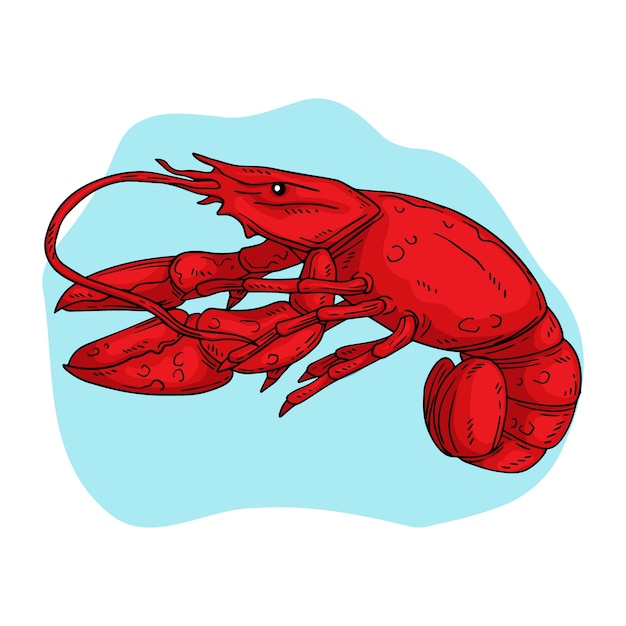This is a cartoonish, vector-style digital drawing of a red crawfish, though it also resembles a lobster. The crawfish is positioned against a light blue background, making it look somewhat like a sticker. The drawing features thin black line art with detailed shading in three tones of red to highlight the body. The crawfish has a thick body, a small curled tail, and is facing left. Its distinct features include two large claws, six smaller legs (three on each side), and a white beady eye outlined in black. Additionally, it has one prominent tentacle and smaller round knots scattered over its body, enhancing its textured appearance. The artistic style is simple yet detailed, employing thin black outlines and embellishments like stripes and half-circles to enhance the overall image.